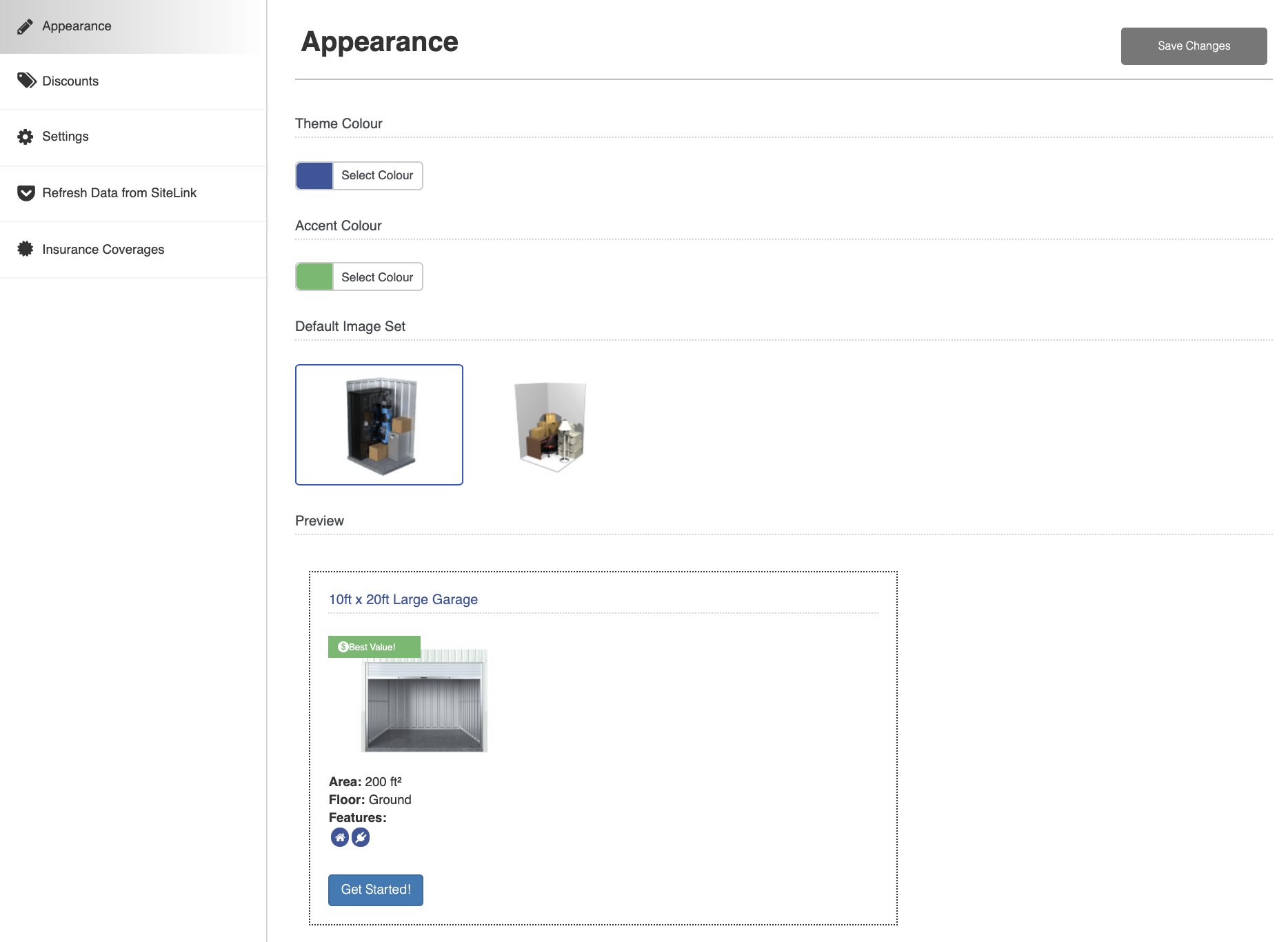Screenshot of a computer screen displaying a settings page from a garage organization design builder. The interface is segmented with five tabs on the left: Appearance, Discounts, Settings, Refresh Data from Site Link, and Insurance Coverages. The selected 'Appearance' tab reveals various customization options, including Theme Color, Accent Color, Default Image Set, and a Preview section. The preview showcases a 10 feet by 20 feet large garage with detailed views of the area, floor, and features, indicating comprehensive design capabilities for organizing and arranging garage spaces. A "Get Started" button is also visible, suggesting an interactive element for users to begin their design process.